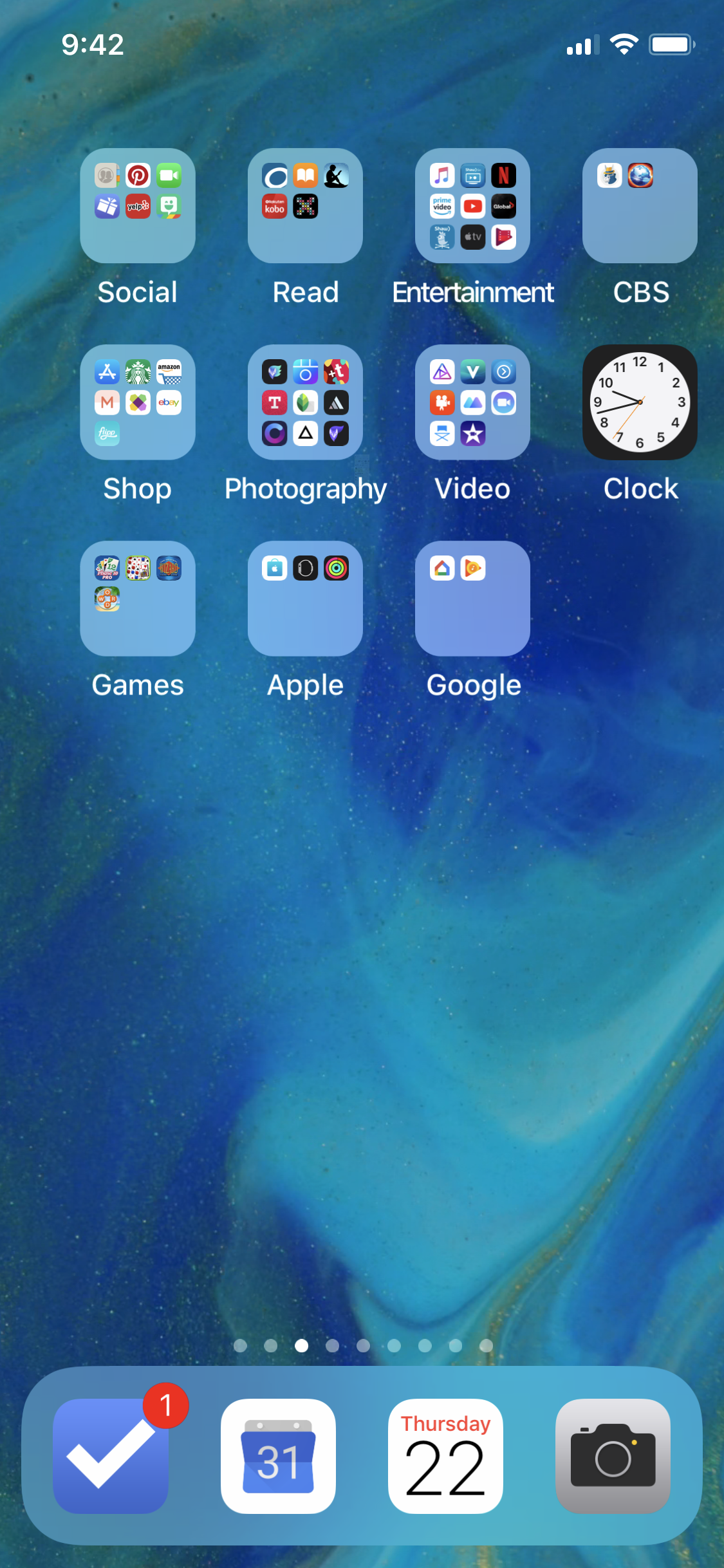The image depicts a smartphone's home screen with various app folders and icons organized in a grid layout. At the top left corner of the screen, the time is displayed as 9:42. Adjacent to the time are indicators for cellular signal strength (three bars and a 4G symbol), Wi-Fi connection, and a fully charged battery.

Below the status bar, several app folders are visible. The first folder is labeled "Social" and contains six icons. The next folder is "Read," featuring four book-themed icons. Following that is the "Entertainment" folder. Next is the "CBS" folder, which contains two icons. The "Shop" folder includes seven icons. The "Photography" folder is populated with nine icons, while the "Video" folder contains eight icons.

There is a separate app icon for the Clock, represented by a black square with a clock face showing the hour hand between eight and nine.

Further, there is a "Games" folder that holds four icons and an "Apple" folder with three icons. The "Google" folder shows two icons.

At the bottom of the screen, nine dots indicate the user is on the third page of the home screen. Directly above these dots, there is a row of fixed icons:
1. A large blue square with a white checkmark and a red notification badge in the top right corner.
2. A white square displaying the number 31.
3. A white square with red text showing "Thursday" and the number 22 below it.
4. A camera icon centered within a white square.

This arrangement on the screen highlights the user's organized method of app management and provides a glimpse into their preferences and frequently used applications.